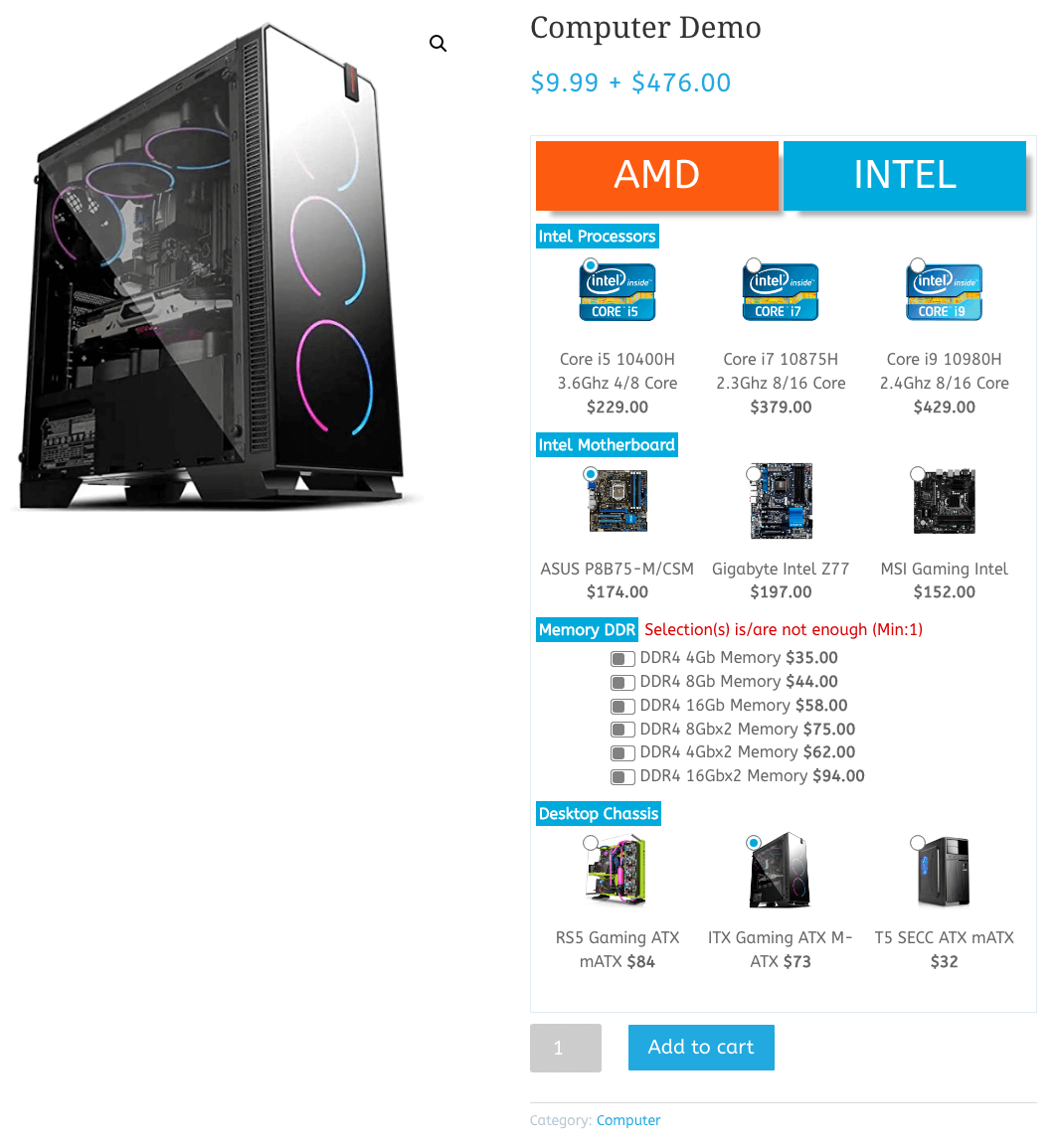The screenshot appears to be from a computer hard drive sales page. At the top of the page, there's a header labeled "Computer Demo," with pricing details stating "$9.99 plus $476." The layout includes a right-hand sidebar and a central image displaying a computer shell on the left. The sidebar on the right offers various components for purchase. 

The components are categorized and listed as follows:
- At the top of the sidebar, there are red and blue rectangles with white text indicating processor brands: "AMD" in red and "Intel" in blue. Currently, Intel is selected.
- Beneath the processor options, there's a selection of processors available for purchase.
- The next section lists different motherboards.
- Following that, there are memory size options for the potential builds.
- At the bottom of the sidebar, there are selections for desktop chassis.

At the very bottom of the page, a blue "Add to Cart" button is prominently displayed, allowing customers to proceed with their customized computer build.

This detailed interface effectively guides users through the process of assembling their own computer by selecting individual components from the provided categories.